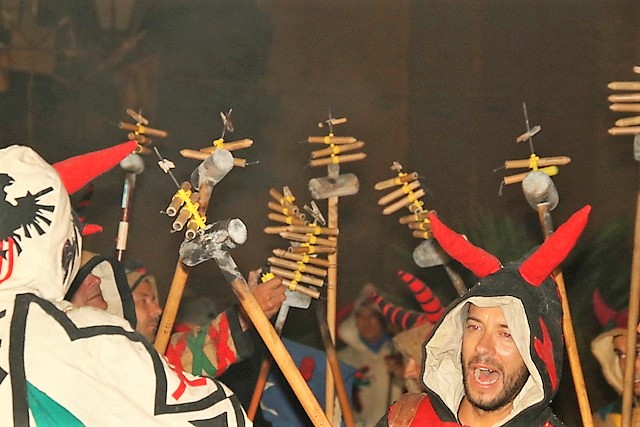The image depicts a vibrant festival scene, centered on a man with a distinctively clear face on the right. This man, possibly of Arab descent, sports a black beard and is seen with his mouth open in an expression of celebration. He wears a black hood adorned with striking red horns, with a hint of white fabric lining the inside. A portion of his shoulders is visible, and he dons clothing with red and black elements, and a notable brown patch on his right shoulder.

To the left, another figure stands with their back to the viewer, cloaked in a white robe with intricate black markings on the hood and shoulders. His attire also features red and green accents, adding to the festive color palette.

In the background, a larger group of men dressed in similar hooded cloaks, many with black, white, and brown patterns, lift wooden sticks into the air. These sticks have mallets or hammer-shaped cylinders attached at the top, secured with yellow strings. Some sticks appear to have small wooden tubes or objects resembling fireworks attached to them. The men in the background hold these sticks at slight angles, contributing to the dynamic energy of the scene.

The background is dimly lit, with a light source providing partial illumination to the four men in the foreground. The upper part of the image reveals an indistinct building structure and hints of green plants. The overall low-light setting, combined with the celebratory postures and vivid costumes, suggests a festive event brimming with cultural significance and communal joy.